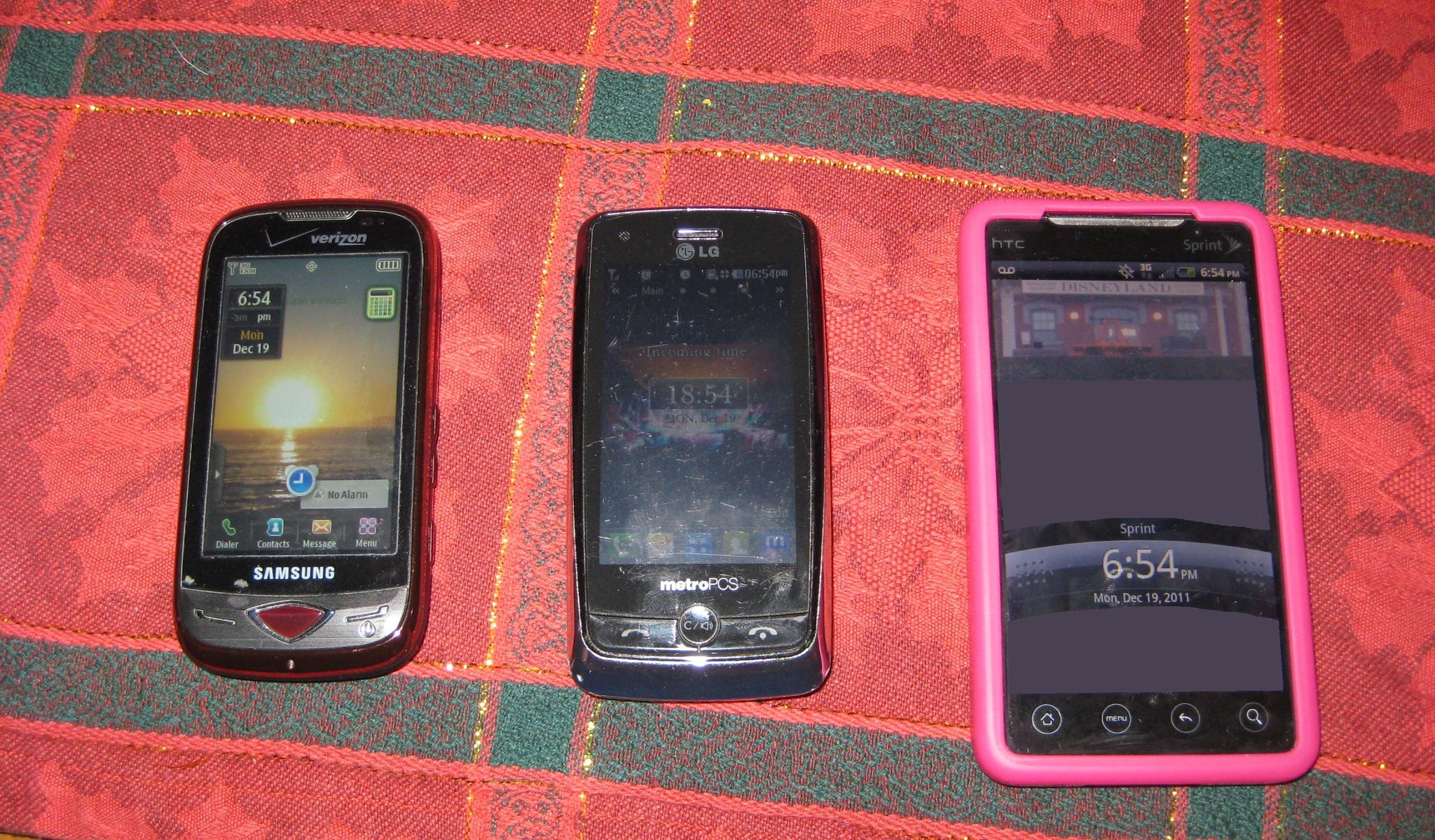This horizontal rectangle photograph features three aged mobile devices arranged on a fabric-covered flat surface. The fabric background is predominantly red with intersecting green and lighter red stripes forming square patterns, each accentuated by gold trim. Within these squares lies a subtle light flower pattern. The primary objects in the image are three smartphones, displaying visible signs of wear.

The leftmost device is a Samsung phone with a physical keyboard revealed by its sliding mechanism. It prominently displays the brand name "Samsung" at the bottom in white letters. Positioned in the middle is an LG smartphone marked by white lettering reading "LG" at the top and "Metro PCS" at the bottom on its screen. The rightmost device appears to be the largest, enclosed in a pink protective case, and indicates the time "6:45 p.m." in white letters on its center screen. This device is identified as an HTC phone under Sprint service and is fully touch screen.

The entire setting suggests the fabric may be a bedspread or couch material, hinting at a casual and domestic environment for the portrayed items.